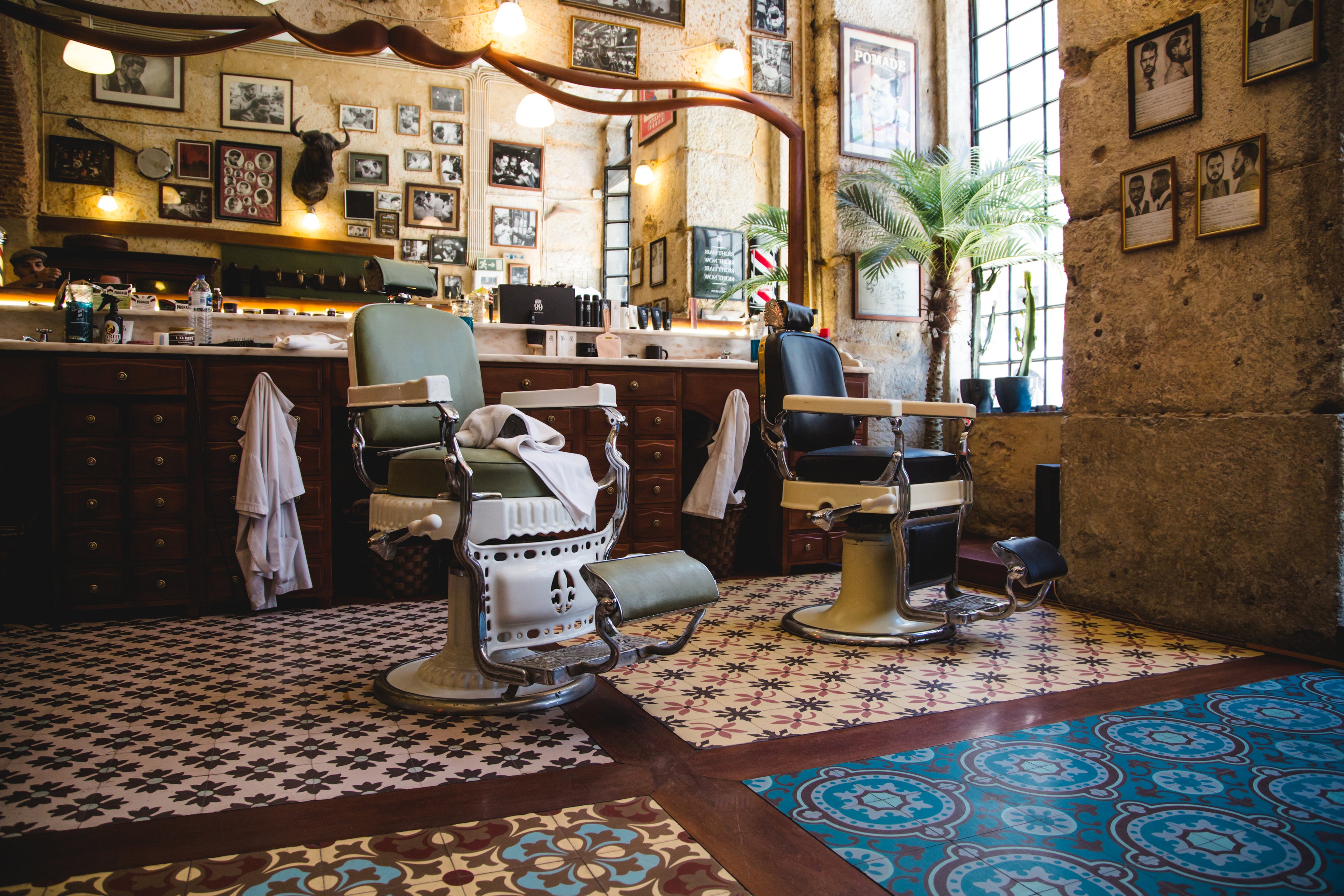The photograph captures a vibrant barbershop setting with two prominent barber chairs situated side by side. The chair on the left displays a mint green hue with a crumpled towel draped on its seat, while the chair on the right comes in dark tones of black or dark blue, accented with gold. These chairs rest upon and face a very intricate floor featuring blue, tan, and floral patterns segmented by brown, wood-like tiles.

Behind the chairs stands a long glass mirror, topped with a distinctive wooden mustache carving. A matching wooden dresser beneath the mirror holds numerous barbering tools, surrounded by jackets hanging on its drawer knobs. To the right, a tall, large window bathes the room in natural light, and flanking this window are lush green plants, including two cacti and a potted palm tree.

The room is decorated with various forms of artwork, photographs, and posters. The brown concrete wall on the left hosts several framed pictures, while the mirror reflects additional artwork on the opposite wall along with quirky items like a banjo and a stuffed animal head. The atmosphere of the barbershop is further energized by the presence of bright ambient light fixtures throughout the space. No people are visible in this image, leaving the colorful and detailed environment as the focal point.